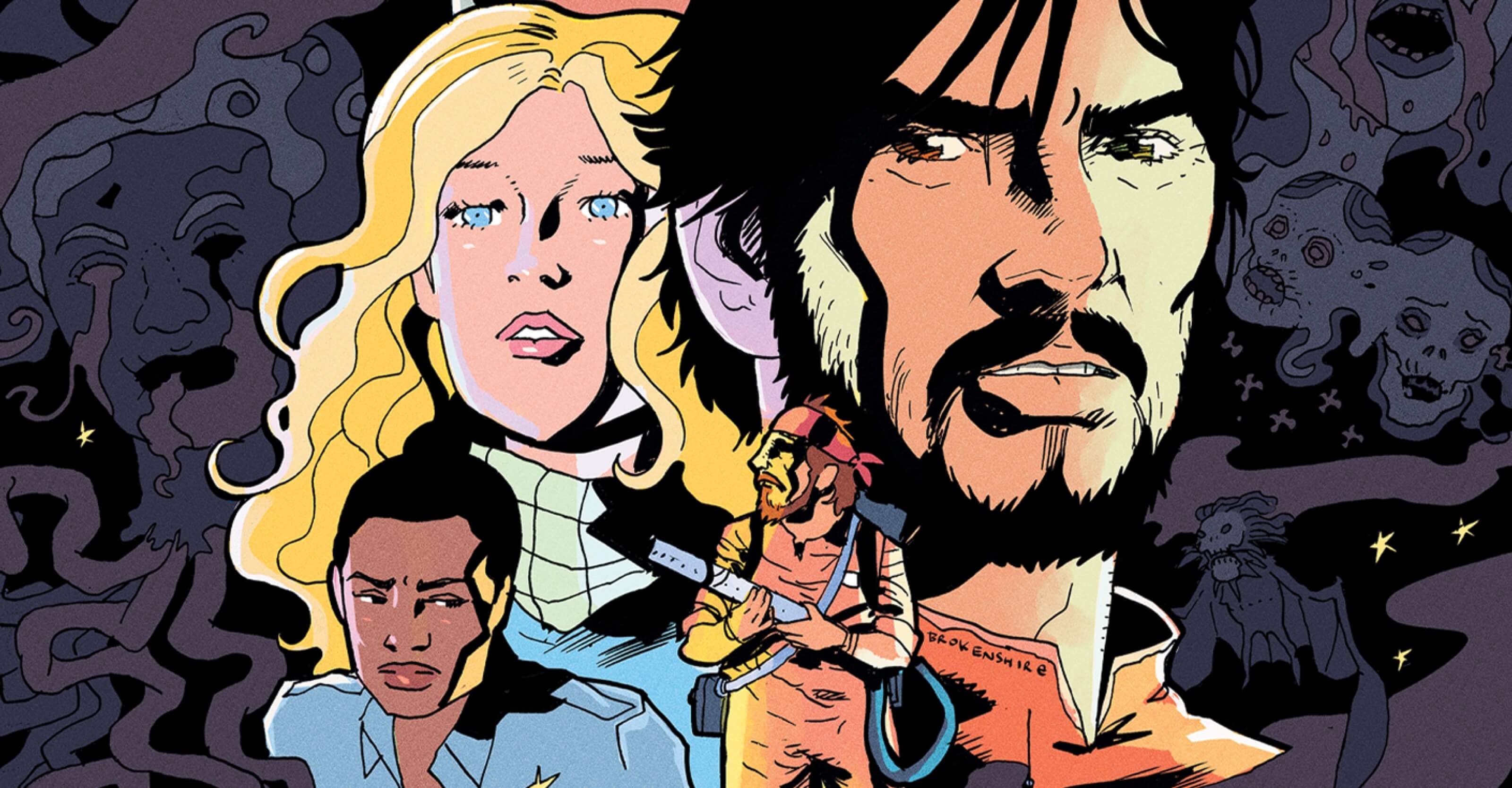This comic illustration, signed "Brokenshire," depicts four distinct characters against a haunting background filled with dark gray and black, featuring deformed faces and skeletal, winged creatures. The main male character, positioned on the right, has black hair and a thick beard and goatee, and he wears an orange suit with a turtleneck. The name "Brokenshire" is visible on his collar. Beside him is a young blonde woman with blue eyes, dressed in a blue uniform and a beige turtleneck, appearing scared and horrified. An African American man with a short crew cut and a blue uniform, partially unzipped to reveal a turtleneck, stands in front, bearing a star on his lapel. Another male character, resembling a Ghostbuster, wears a backward hat, has a beard and mustache with obscured eyes, and carries a device with a tube on his back and a gun-like apparatus. The chilling ambience is heightened by floating, winged skulls and a face with melting eyes, all enveloped in a ghostly, shadowy backdrop illuminated by four yellow stars.